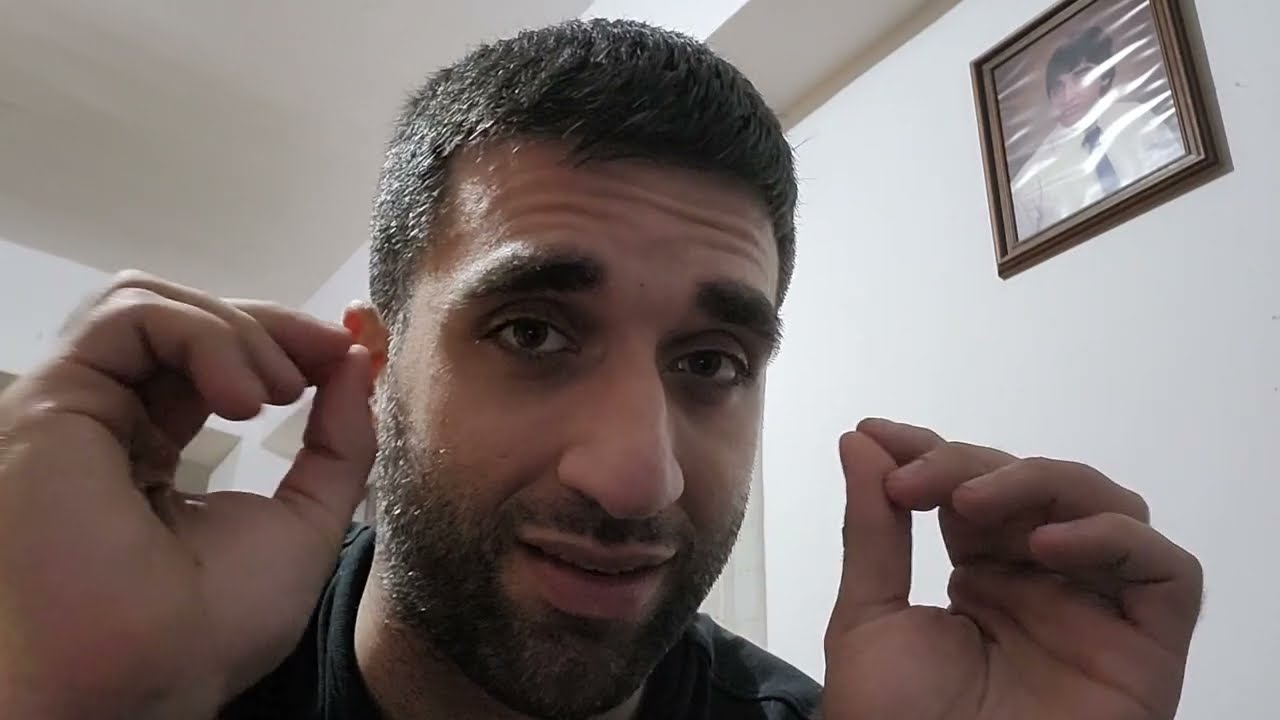The image is a close-up photograph of a man who appears to be in his late 20s to early 30s. He has short, cropped black hair, a black beard, and notably thick eyebrows. His complexion is olive, suggesting he might be of Middle Eastern, East Asian, Indian, Pakistani, or Arab descent. The man is positioned slightly to the center-left of the frame, facing the viewer directly, with a somewhat incredulous expression as if to say "really?" 

His hands are raised beside his head, with his thumbs and index fingers forming small "O" shapes, possibly indicating a gesture commonly used while talking. He is wearing a black shirt or t-shirt and seems to be inside a white-walled room, possibly in a house or bedroom. 

In the upper right corner of the image, behind the man, there is a white wall with a framed picture. The portrait appears to show another man, likely a younger version of the man in the foreground, dressed in a white shirt and blue tie, resembling a formal or school photo. The interaction between the man and the camera, combined with the setting and background details, creates a detailed and evocative scene.